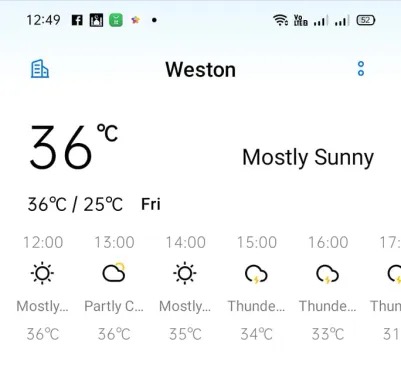A detailed caption could be:

"Captured from a cell phone screen, the image displays the device's current time at 12:49 PM. Various icons are visible at the top: a green square, a Wi-Fi signal icon showing partial strength, and a battery icon indicating a 52% charge. On the left side, there's an icon resembling two diagonal buildings. Centrally located on the screen is the word 'Weston,' written with a capital 'W' followed by lowercase letters. Two small blue circles follow the label. Below this, on the left side, the temperature is displayed as '36°C,' with a slash marking '36°C / 25°C,' likely indicating the high and low temperatures for the day. To the right, 'Mostly Sunny' is noted. Further details on the forecast are shown below, with hourly temperatures listed for 12 o'clock through 17 o'clock. Starting from 36°C at 12 PM, the temperature gradually declines through the hours: 35°C at 2 PM, 34°C at 3 PM, 33°C at 4 PM, and 31°C at 5 PM. Weather icons, presumably clouds, accompany these hourly updates."